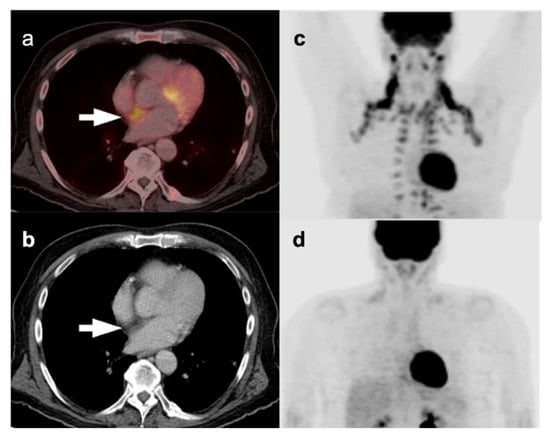The image consists of four distinct medical scans, each labeled with lowercase letters 'a,' 'b,' 'c,' and 'd' arranged in a quadrant layout. The top left quadrant, labeled 'a,' appears to show a brain scan with some form of discrepancy highlighted, and includes an arrow pointing to the area of concern. Directly to the right, in the top right quadrant labeled 'c,' is an x-ray of a person's abdomen with a noticeable black spot near the stomach. The bottom two quadrants feature, to the left labeled 'b,' a grayscale brain scan, similar to 'a', and to the right, labeled 'd,' another x-ray showing significant dark spots in the chest area, near the heart and brain. This comprehensive collection of scans presents a detailed view of different parts of a human body, emphasizing notable discrepancies and abnormalities.